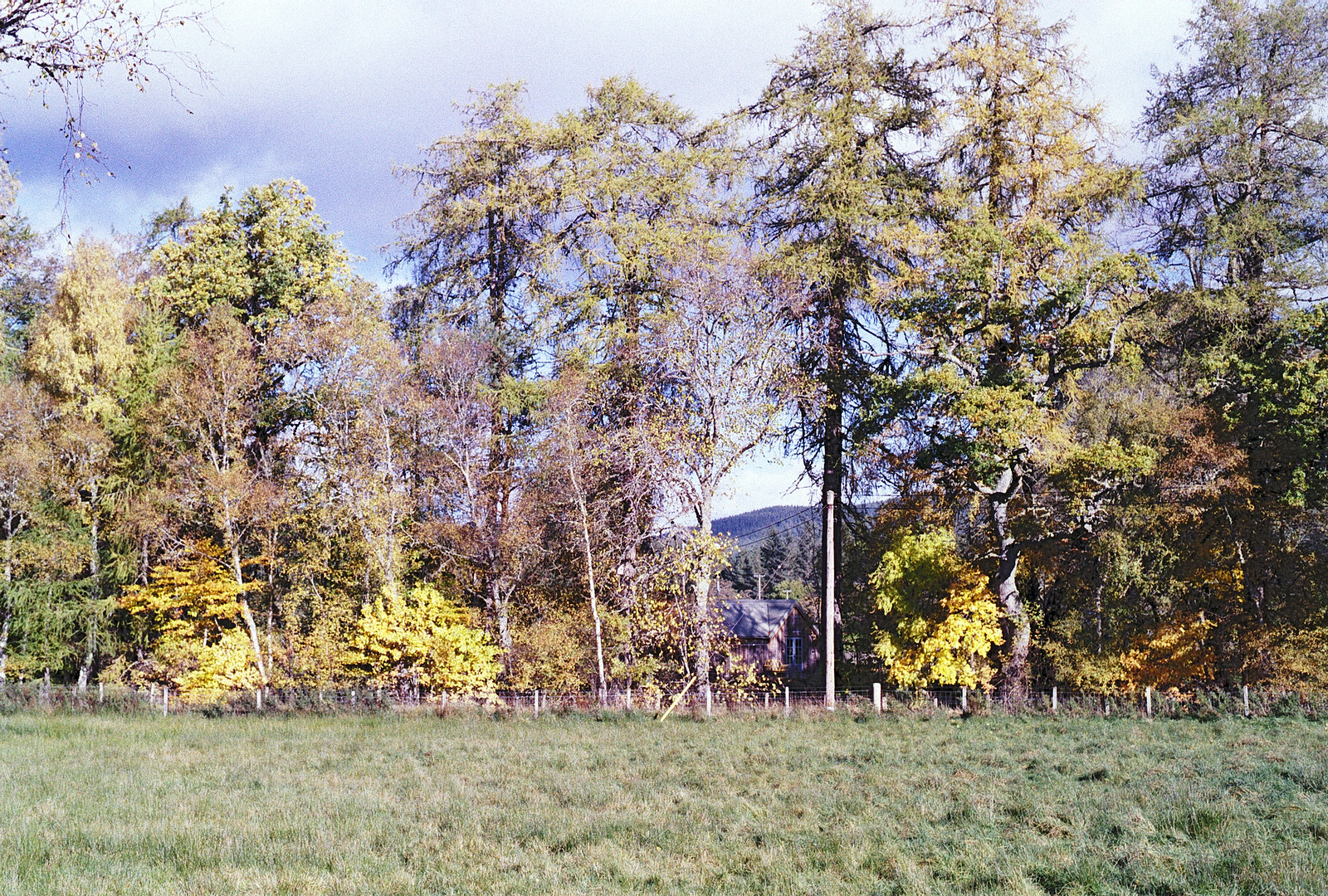The image captures a picturesque field bordered by a wood rail and wire fence, with a blend of green grass on the far right side transitioning to patches of dried-up grass on the left. The scene is adorned by a variety of trees, some lacking leaves while others display vibrant yellow foliage, especially towards the bottom. Among these trees, two notably tall ones stand in the center alongside another prominent tree on the far right. The backdrop features a mix of pine trees interspersed with smaller aspens closer to the fence. Above, the sky is mostly cloudy with shades of white and gray, subtly interspersed with hints of blue. In the distance, rolling hills form a gentle skyline, and a house or cabin with a gray roof is nestled amongst the trees, offering a rustic charm. The field, devoid of any visible animals, appears primed for pasture land, with its serene and open landscape extending into the horizon.